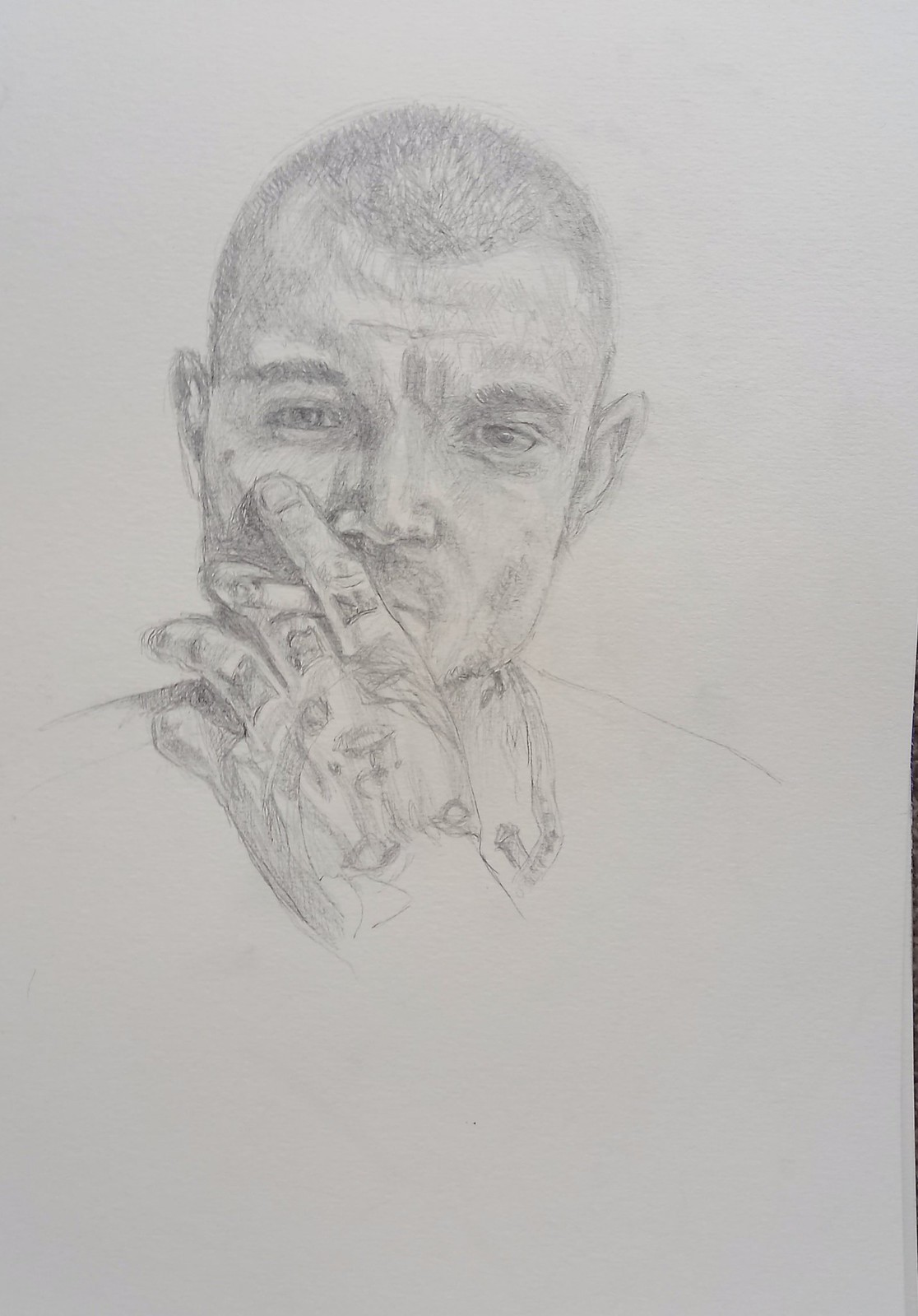This highly detailed pencil drawing depicts a man with his left hand positioned thoughtfully against his face. His thumb rests under the right side of his chin, while his index finger is placed gently beneath his right eye. The rest of his fingers are naturally contoured along the side of his face. The middle and ring fingers are slightly bent, maintaining a normal distance from each other, with the pinky finger close by.

The man sports a short, military-style haircut and a faint beard, suggestive of a five o'clock shadow. His ears are subtly pointed, adding a distinct feature to his appearance. He holds a cigarette between his index and middle fingers, the smoke curling softly into the air.

Intricately inked on his hand is a tattoo of a woman's face. The tattoo extends from his middle finger towards his wrist, showcasing detailed features including lips, a nose, and two eyes, all exquisitely rendered within the confines of the hand tattoo. This drawing captures both the rugged, thoughtful demeanor of the man and the artistic intricacy of the tattoo, making it a compelling visual narrative.